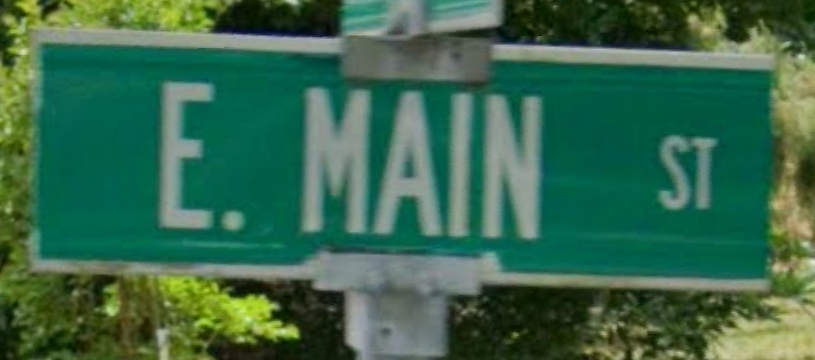This image presents an extreme close-up of a green street sign for "E. MAIN ST" affixed to a metal pole via a robust mounting bracket. The sign, positioned horizontally and stretching wide but not very tall, features bold, white, capitalized lettering. A thin white metal slot runs across the bottom and top edges of the sign. The mounting bracket is a prominent aluminum structure with a square pattern and metal clamps securing the sign to the pole. Above it, the lower part of an adjacent sign is visible, though its details are indistinct. In the background, various trees and vegetation are visible, including a light green tree one-third from the left, a dark green tree spanning across the middle, and another light green tree towards the right near a patch of green ground. Some of these elements are brightly lit, while others remain in shadow, adding depth to the scene.